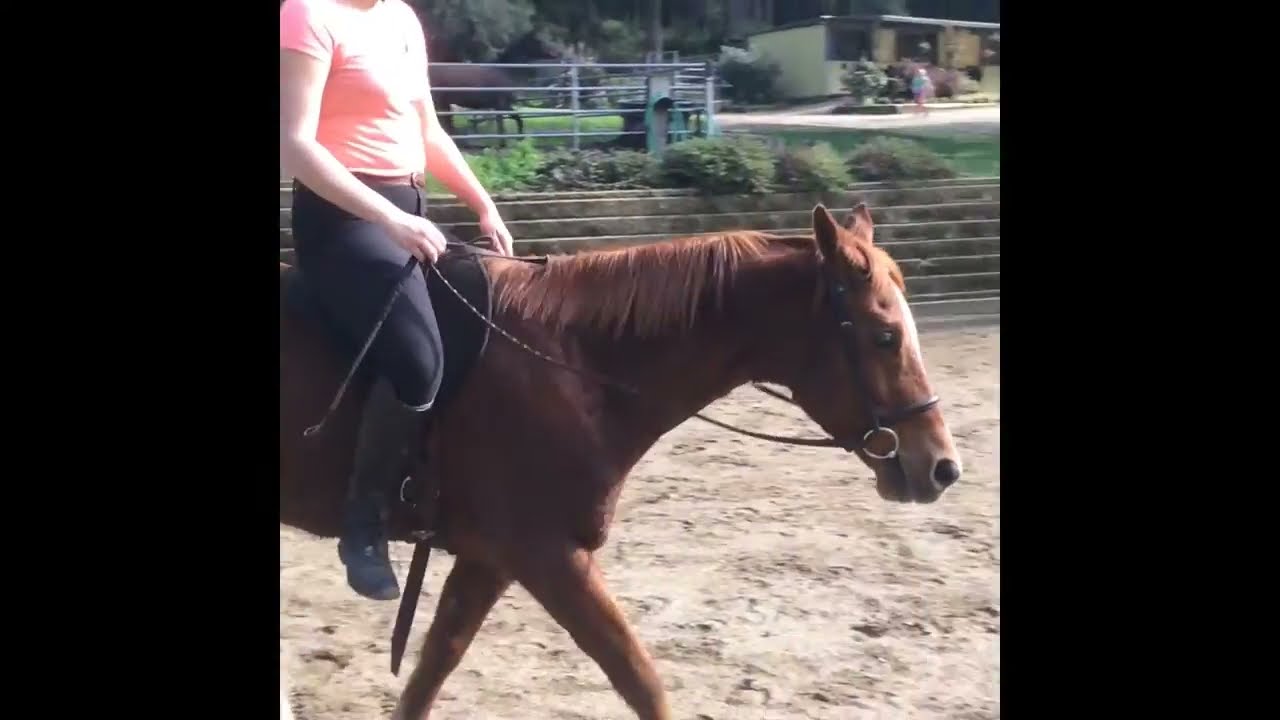In the image, a woman is riding a brown horse with a white stripe down its forehead. The photo, which focuses more on the horse than the rider, cuts off the rider's head, showing only her torso and legs. She is dressed in dark pants, black leather boots, and a pink short-sleeve shirt, and holds a black whip down by her side. The horse has a black saddle, is adorned with rings and leather straps around its head, and has its ears facing backward while walking with its head lowered. The front legs of the horse are in a triangular pattern, indicating movement on a light sandy ground. The background features several details: a gray brick wall, green bushes, and an enclosure with fences. Further back, another horse can be seen in a separate fenced area. On the top right, there's a small building, possibly a stable, with a blurred figure walking beside it. The overall scene gives a clear view of a typical equestrian setting with various elements of greenery and a sandy pathway.